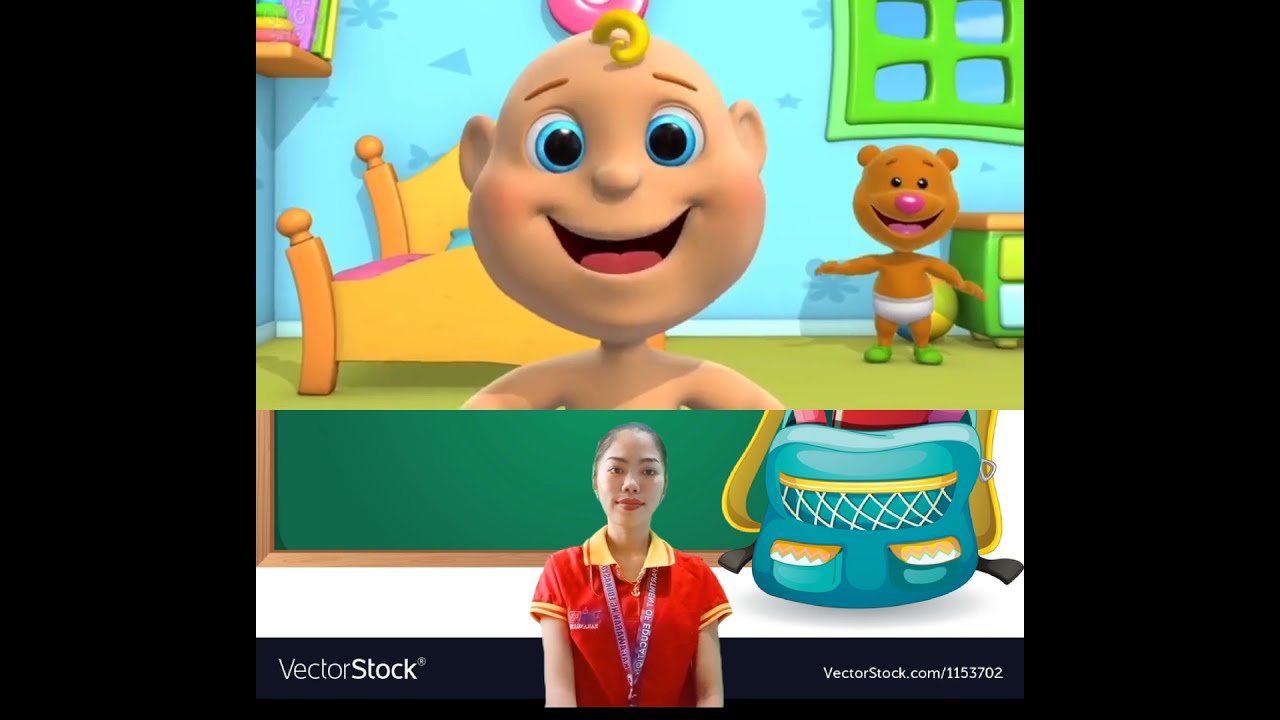The image is a wide rectangular split-screen featuring two distinct scenes. At the top, a fully animated, CGI-generated cartoon scene depicts a smiling baby with blue eyes and a tuft of blonde hair. Behind the baby, a teddy bear in underwear smiles, set in a vibrant bedroom with bright blue walls, a green window revealing a blue sky, a bed, a shelf, and a small stand. Various colors fill the scene, creating a lively and detailed environment.

At the bottom of the image, a real-life Asian woman stands facing forward. Only her torso and head are visible. She has light skin, her hair is pulled back, and she wears red lipstick. Her attire includes a red short-sleeved polo shirt with yellow stripes at the sleeves and collar, and a pink and purple lanyard around her neck. Behind her, there is a chalkboard and the partial image of a small backpack. Both sides of the image are bordered by black rectangles, cropping it into a neat frame. The watermark "Vectorstock" is visible at the very bottom, along with the URL "Vectorstock.com/1153702" on the bottom right.